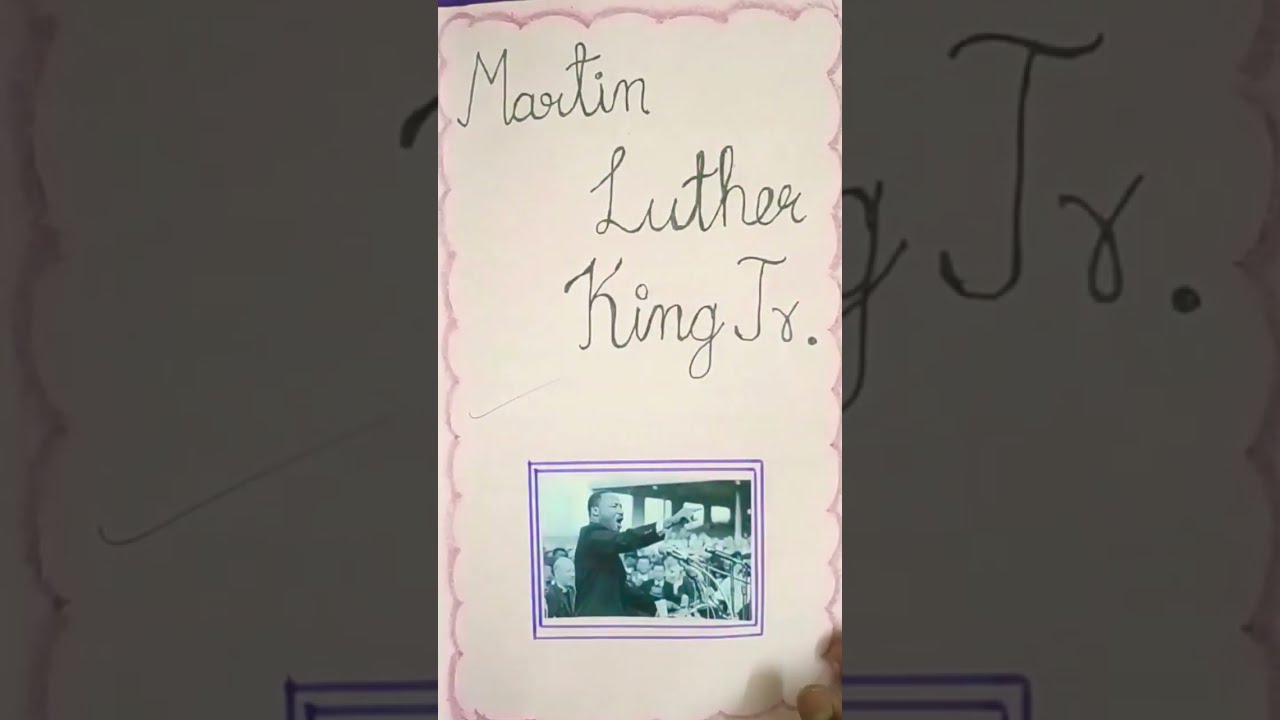The image depicts a piece of paper with handwritten, cursive text that reads "Martin Luther King Jr."—with "Martin" on the top line, "Luther" in the middle, and "King Jr." on the bottom. Below the text is a black-and-white photograph of Martin Luther King Jr. at a civil rights rally, where he is seen wearing a suit and speaking passionately into numerous microphones, his hand raised with a pointed finger. The paper itself is pinkish in color and is bordered by a cloud-like, pink outline. The main photo is centrally placed, flanked by fragmented, zoomed-in shots of the same image on either side. These fragments are enclosed within thin, purple rectangular lines, adding to the layered complexity of the composition. The image gives an impression of celebrating Martin Luther King Jr.'s legacy, possibly created by a young student, and carries a sense of reverence and historical significance.